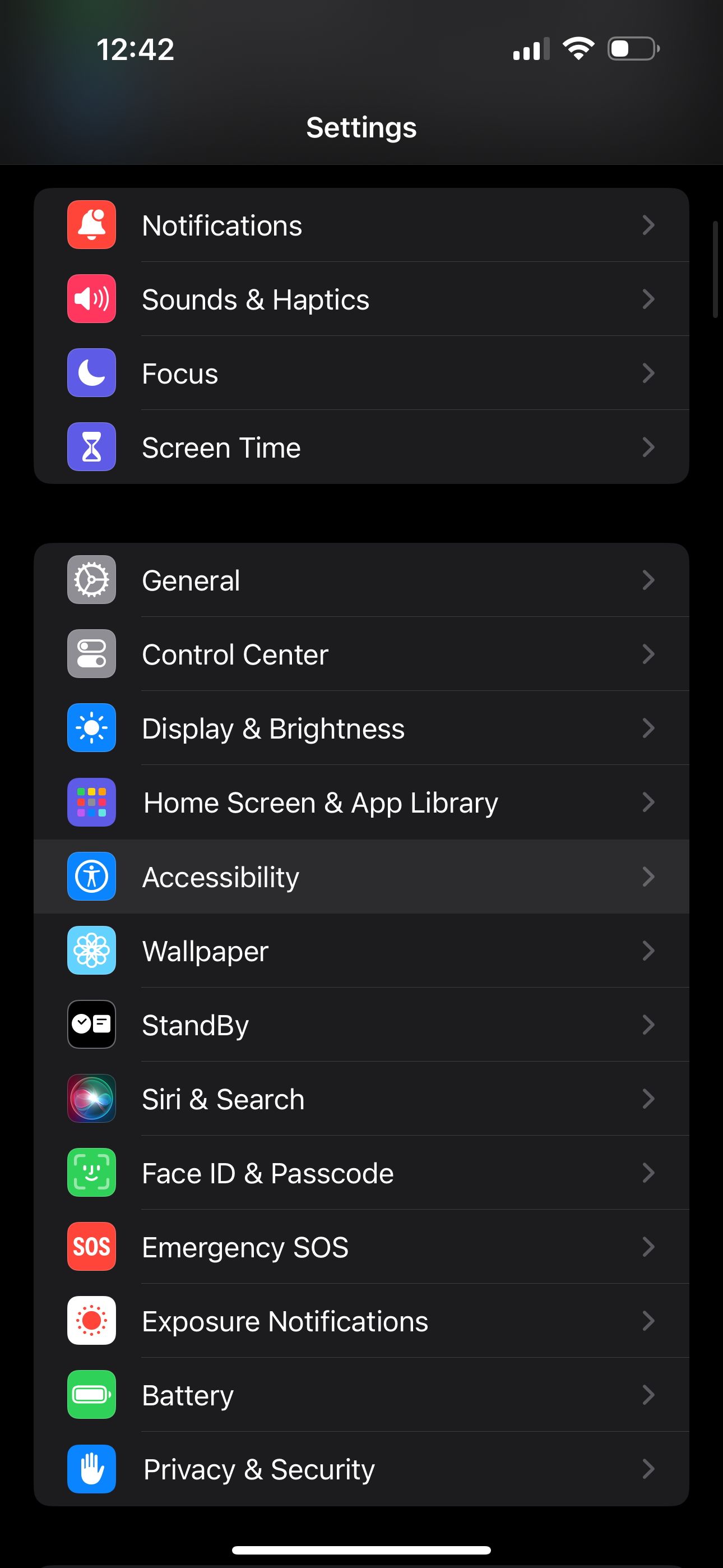This is a detailed screenshot of a mobile phone application displaying the "Settings" menu. The interface features a dark grey header at the top. On the left side of the header, in white text, it reads "12:42". A faint greenish glow is also visible over this text. Moving to the right, the header includes an icon indicating mobile signal strength, with three full white bars and one dark grey bar on the right. Next to this, there is a white Wi-Fi icon, followed by a white battery icon showing approximately 33% charge.

Centralized at the bottom of this header in white text is the word “Settings.” Below the header lies the main body of the page, set against a black background. Two prominent pop-up areas with dark grey backgrounds and rounded corners stand out. The first pop-up is smaller, while the second one is significantly taller. Both pop-ups are divided into several sections by thin light grey lines running almost, but not entirely, from the right edge to the left—approximately 90% of the way.

Each section contains an icon on the left. These icons are square with rounded corners, featuring a colored background and a specific symbol on top. Adjacent to each icon, to the right, is a line of white text.

The first, smaller pop-up includes the following sections (from top to bottom):
1. Notifications
2. Sounds & Haptics
3. Focus
4. Screen Time

The second, taller pop-up includes a more extensive list of sections (from top to bottom):
1. General
2. Control Center
3. Display & Brightness
4. Home Screen & App Library
5. Accessibility
6. Wallpaper
7. Standby
8. Siri & Search
9. Face ID & Passcode
10. Emergency SOS
11. Exposure Notifications
12. Battery
13. Privacy & Security

This organized and structured UI provides easy navigation through various settings options on the mobile application.